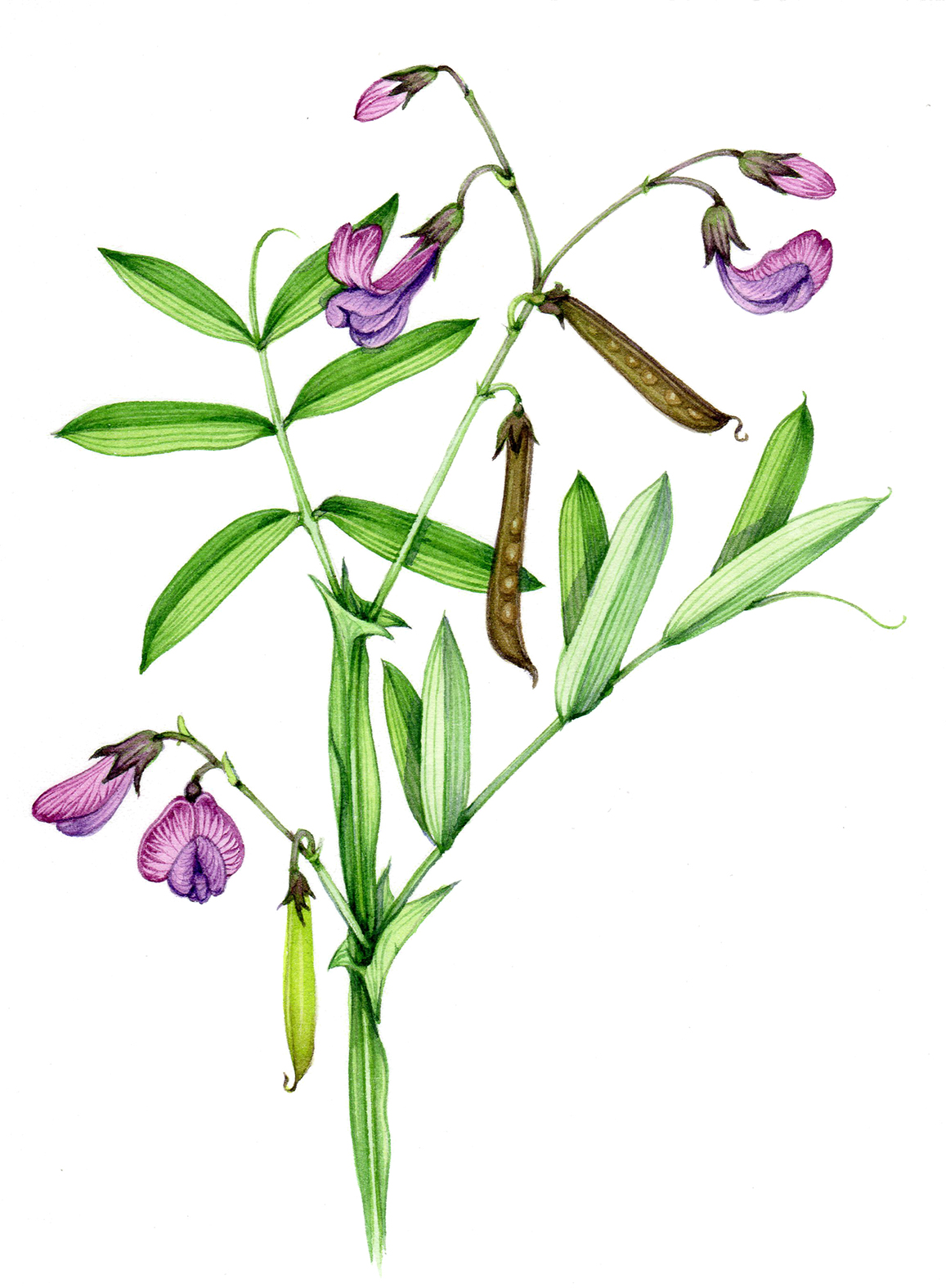This image is a detailed, colored illustration of a plant featuring various elements. The plant has a central green stem with multiple long, vibrant green leaves sprouting from it. On the lower left and upper right sides, small clusters of flowers are visible. These flowers resemble orchids, with some already in bloom while others are budding. There are six flowers in total, with shades ranging from lavender to deep purple, illustrating different stages of blooming.

In addition to the flowers, the plant also has darker yellowish-green and light green pea pods hanging from the stems. Specifically, there are two darker pods and one lighter pod emerging from different parts of the plant. Brown leaves with light brown seeds, resembling little eggs, are interspersed among the green leaves and flowers.

The background of the image is blank and entirely white, which highlights the vivid colors and intricate details of the plant, making it almost pop out of the scene. The entire composition is rich in green and purple hues with touches of brown, creating a harmonious yet simple natural aesthetic.